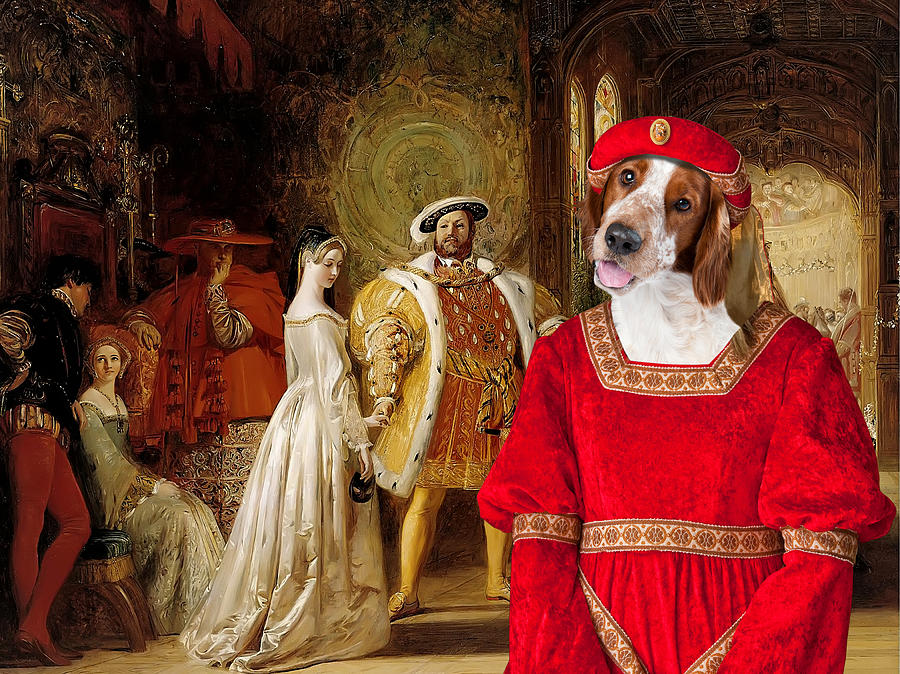The painting captures a lively and humorous royal court scene, with the focal point being a dog, likely a beagle or hound, dressed as a princess. The dog's head, superimposed onto a human body, features long droopy brown ears, a black nose, a pink tongue, and two brown eyes. It wears a meticulously detailed Victorian red dress, adorned with gold trim and an embroidered ribbon around the neckline, waist, and mid-zone of the sleeves. The ensemble is completed with a red princess headpiece resembling a crown.

To the left of the dog stands a grand figure resembling King Henry, a large, imposing man in tights and a majestic coat lined with white fur and accented with red. Next to him is an elegant woman in an ivory dress with gold trim, looking downward. Further left, another man wears a giant red coat and hat, and beside him sits a woman engaged in conversation with someone leaning on her shoulder.

In the background, there are three more figures involved in conversation amidst a richly decorated hall featuring reds and oranges. The scene blends humor and intricacy, with detailed costumes and a playful royal ambiance.